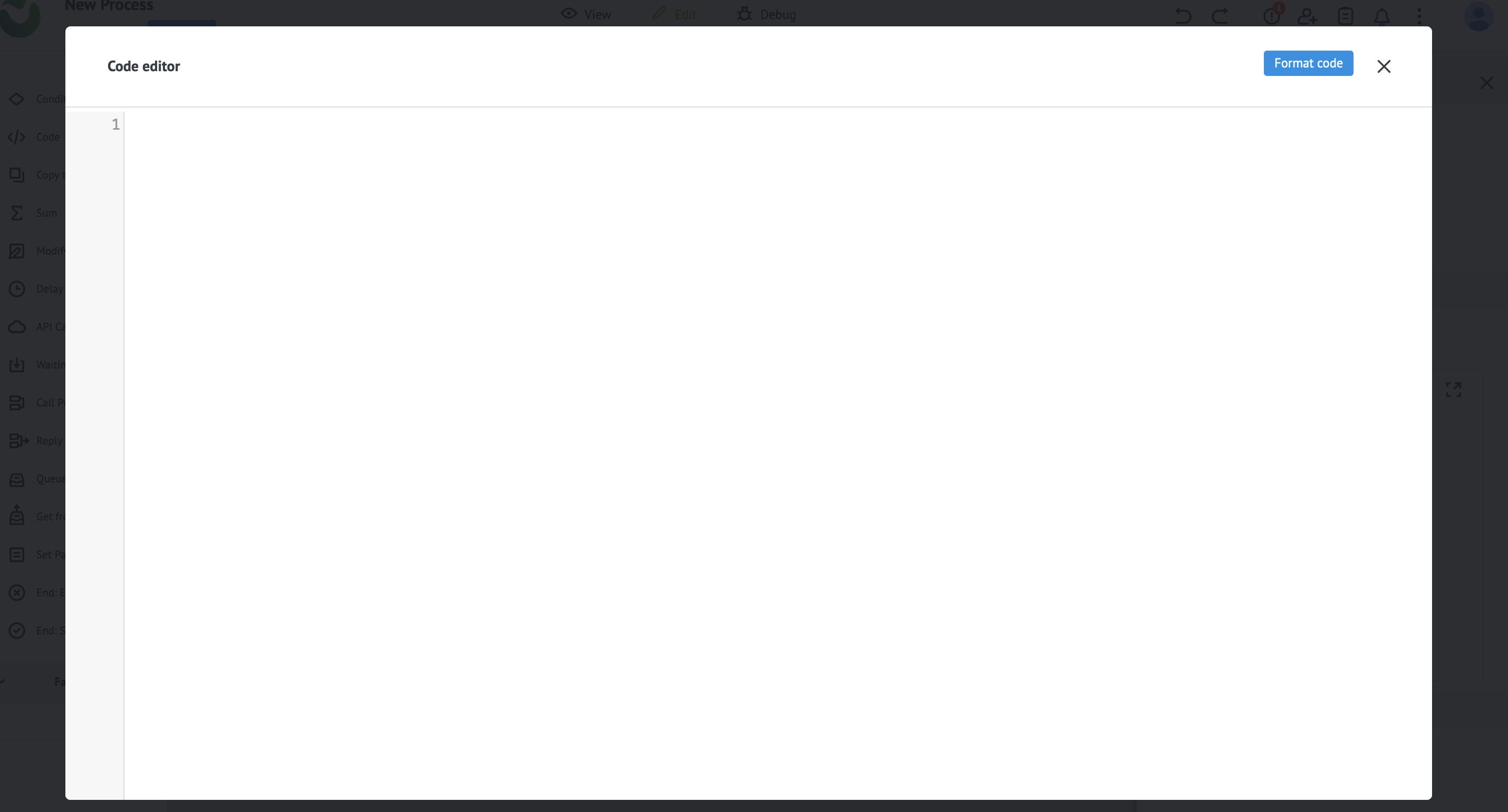The image predominantly features a popping up overlay against a gray background. Central to the image is a white pop-up window labeled "Code Editor" in black text at its upper left corner. A horizontal thin line runs across the pop-up just below this title.

The background elements visible in the interface include various menu items across the top: starting from the left, the word "New Process", followed by "View", "Edit", and "Debug". There are arrow icons representing undo and redo actions. A circular icon with a black border and a white interior contains an exclamation mark, positioned next to a red notification circle with a white number '1'. Beneath these, there's an icon resembling a body shape with a plus sign, a paper sheet icon, an outline of a belt, and three interconnected circles.

On the extreme right end of the interface, a blue circle with an icon of a person appears. The pop-up window features a blue rectangular button labeled "Format" in white and the capital letter F, followed by the word "Code". A black "X" for closing the pop-up is situated at the upper right corner of the white pop-up. Below the thin line within the pop-up, a gray area is present on the left-hand side, displaying the number "1".